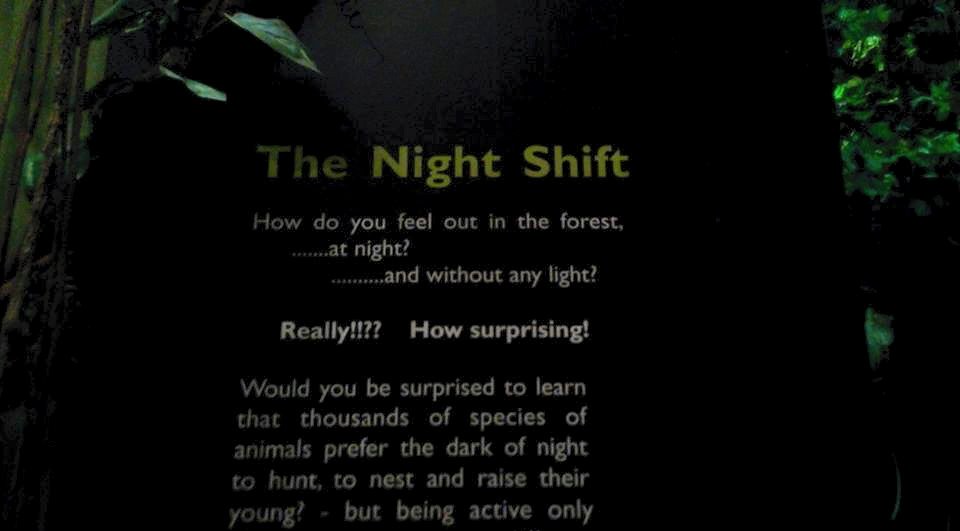In the image, there is a captivating black plaque titled "The Night Shift" in prominent yellow letters, drawing immediate attention. This plaque, possibly attached to a tree or a framework of sticks and set against a backdrop of a dark forest, is designed to educate viewers about nocturnal wildlife. The text begins with an engaging question: "How do you feel out in the forest at night and without any light?" This mysterious and thought-provoking introduction leads into information about the numerous species of animals that prefer the cover of night for activities such as hunting, nesting, and raising their young. Although the full message is partially obscured, the lush greenery and shrubbery surrounding the plaque underscore the forest setting. The ambient darkness along with some subtle lighting enhances the nocturnal theme, effectively immersing viewers in the subject matter.